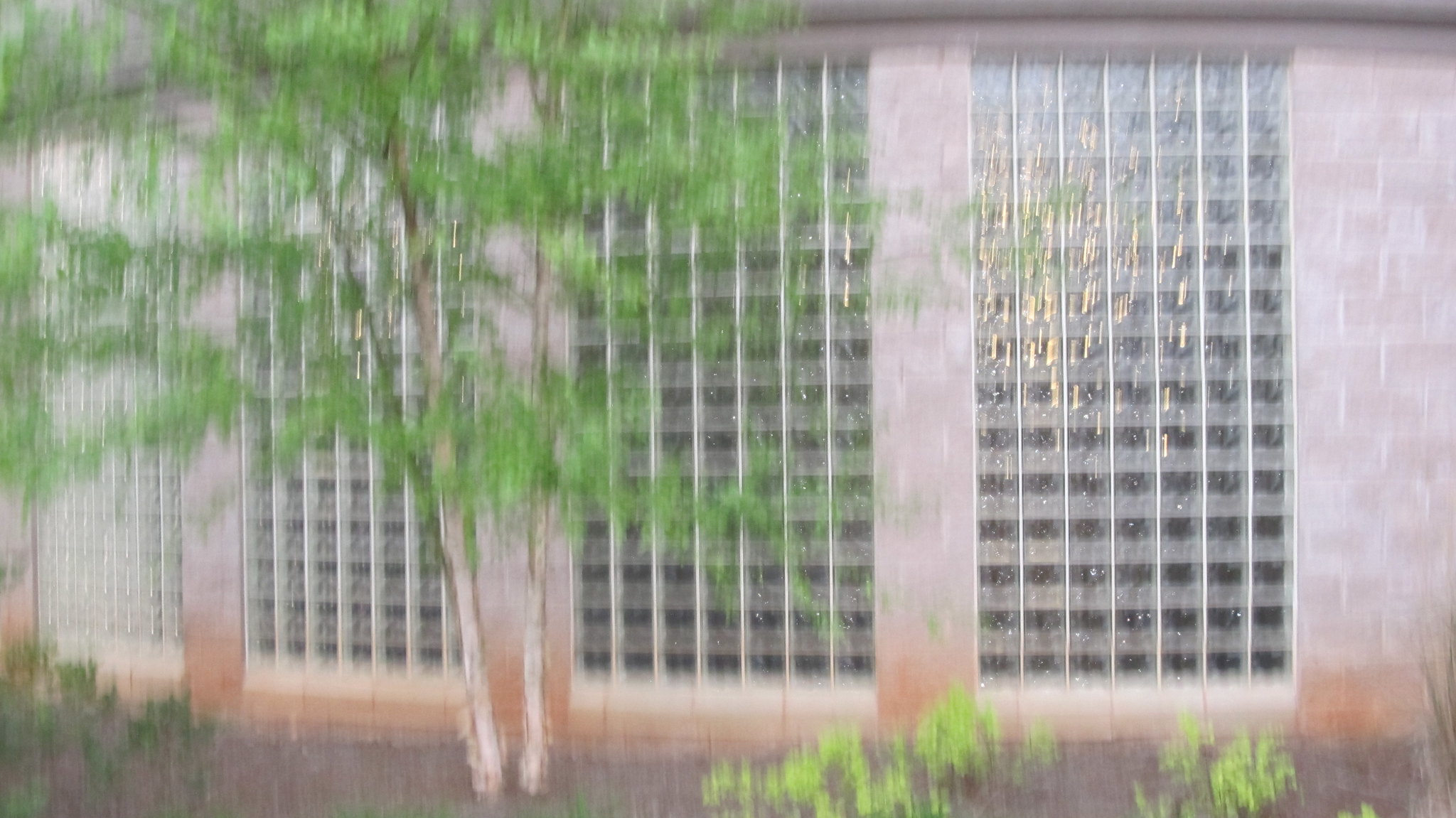This outdoor color photograph, taken during the daytime, features a sparse, brown-barked tree with sparse green leaves dominating the left of the center foreground. The tree stands around one story tall, and its foliage is thin enough to easily see through to the background. Behind the tree, a cinderblock wall is visible, housing four rectangular windows made up of multiple translucent glass blocks that obscure direct visibility. In the foreground, a mostly dirt garden with a few small bushes is visible to the right and left of the tree. The image, though well-lit, is very blurry and contains no text or print.